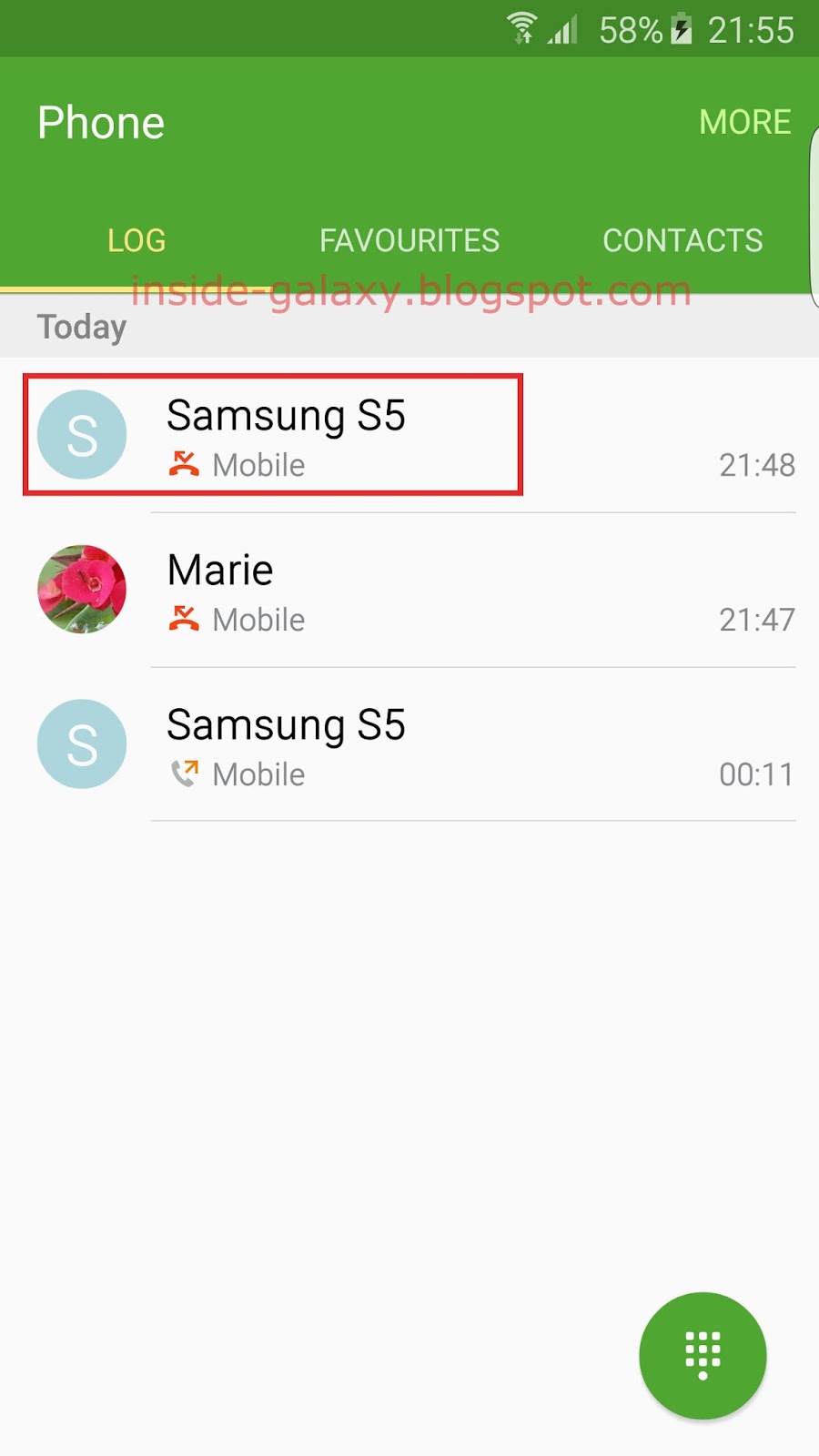The screenshot shows a minimalistic user interface of a smartphone. At the top, a wide green banner spans the screen, with a darker green rectangular section at the very top displaying key status icons. On this darker green section, the Wi-Fi signal icon is visible, followed by three out of four possible bars indicating network strength. To the far right, the battery icon, half-full with a black lightning bolt, shows a charge level of 58%. The time, displayed in white, reads 21:55.

Beneath the status bar, the word "Phone" in large white letters is positioned on the left, and "More" appears on the right in white lettering. Centered below these headings are three options also in white: "Log" on the left, "Favorites" in the middle, and "Contacts" on the right. Just below this green banner, in red letters peeking out, is the URL "insidegalaxyblogspace.com."

On the left side against a muted gray background, the word "Today" is written in black, with three lines of information underneath it, indicating recent incoming calls. Each entry is associated with blue-gray circles containing initials or icons. The first line reads "Samsung S5 mobile" at 21:48. The second entry, next to a circle with roses, is from "Marie" at 21:47. The final entry, next to another blue-gray circle with an "S," notes a call from "Samsung S5" at 12:11.

In the bottom right corner of the screenshot, there is a green circle containing a white square – the button for accessing the phone's dial pad.